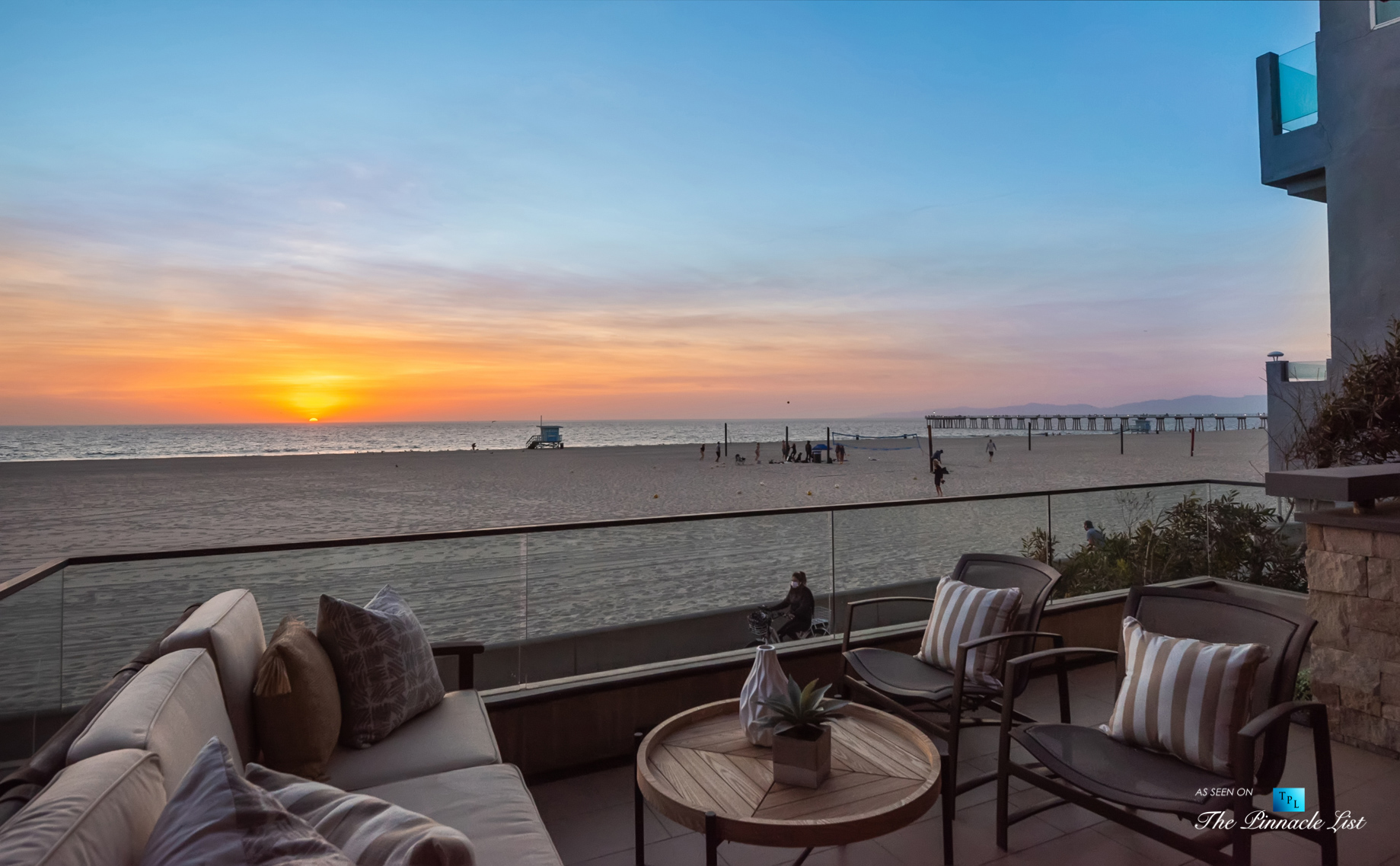On a picturesque patio overlooking the beach at sunset, this square-shaped wooden deck features low glass railings topped with wooden panels. In the bottom left corner, a three-seat outdoor sofa with gray cushions and brown pillows leans against armrests, complemented by nearby brown metal and canvas chairs facing it. A round wooden table with black metal legs stands adjacent, hosting a square planter with a lush green fern and a tiny plant in a white, round planter.

Beyond the patio, the sky displays a gradient from light blue to warm hues of orange and yellow as the sun sets over the horizon. The serene ocean and sandy beach stretch out below, dotted with people enjoying activities like volleyball. A notable pier extends into the water, while lifeguard shacks and multi-story resort buildings line the beach, enhancing the idyllic coastal scene.